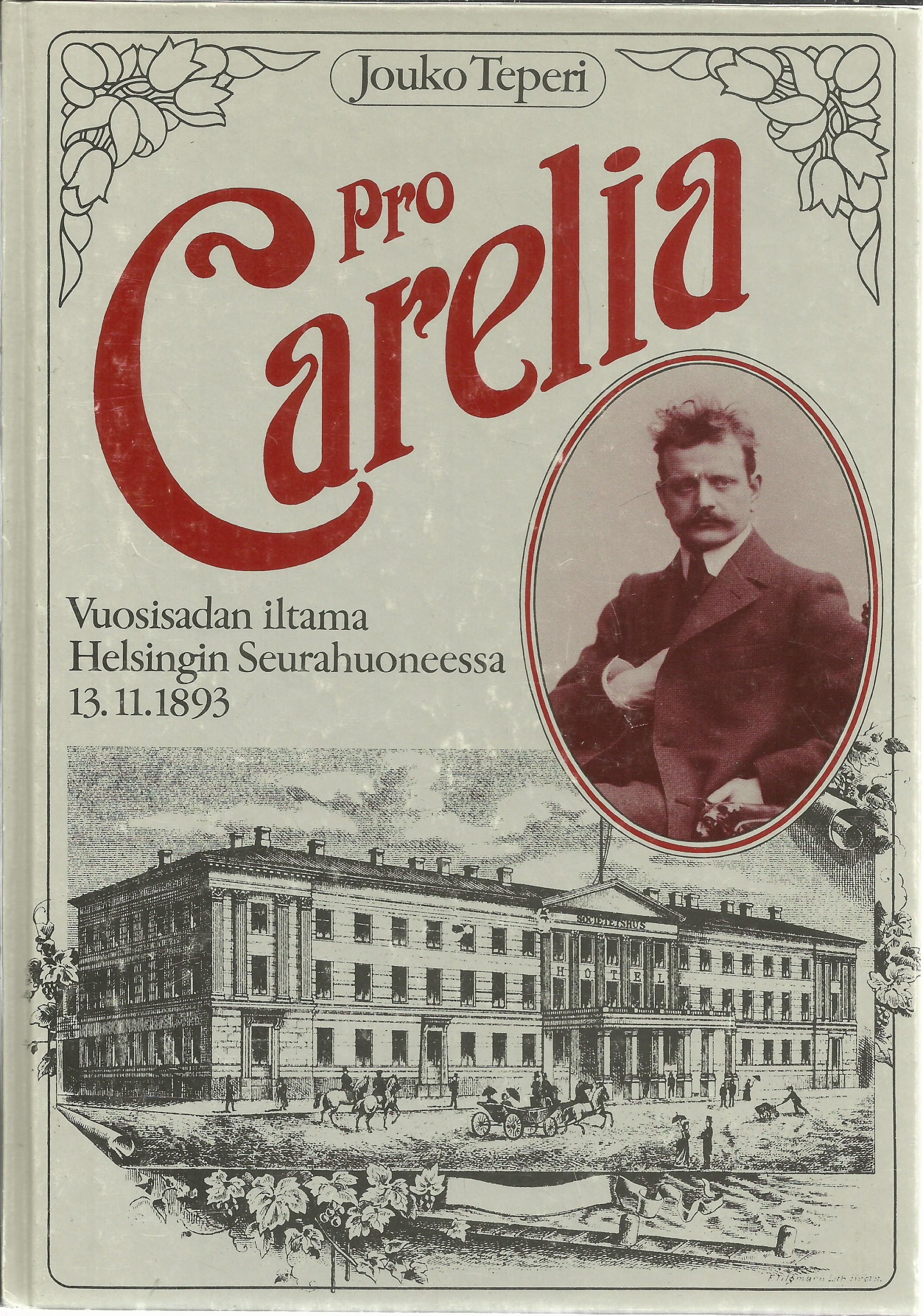The cover of this vintage book is a study in detailed artistry and historical intrigue. Set against a grayish background, the design is striking in its simplicity and complexity. At the top, two words, "Jouko Teperi," possibly the author's name, are stylishly inscribed within a capsule-shaped design, framed by a delicate floral border at each top corner. The border consists of tulip-like flowers, rounded shapes, and outlines of stems and leaves.

Beneath this, the book's title, "Pro Carelia," is prominently displayed in large, bold red letters. Adjacent to the title, a vertical oval frame contains a black-and-white photograph, tinted with various shades of red, of a distinguished gentleman. He wears a suit and tie, his mustache finely groomed, and his wild hair adds character to his composed appearance. His right hand is tucked into the suit’s inner pocket, and he looks contemplatively to his left.

Below this compelling image, a historic scene unfolds, rendered in black and white. It features a hotel with horse-drawn carriages and people bustling about, evoking a bygone era. A date, 13-11-1893, adds a concrete temporal anchor to this evocative cover.